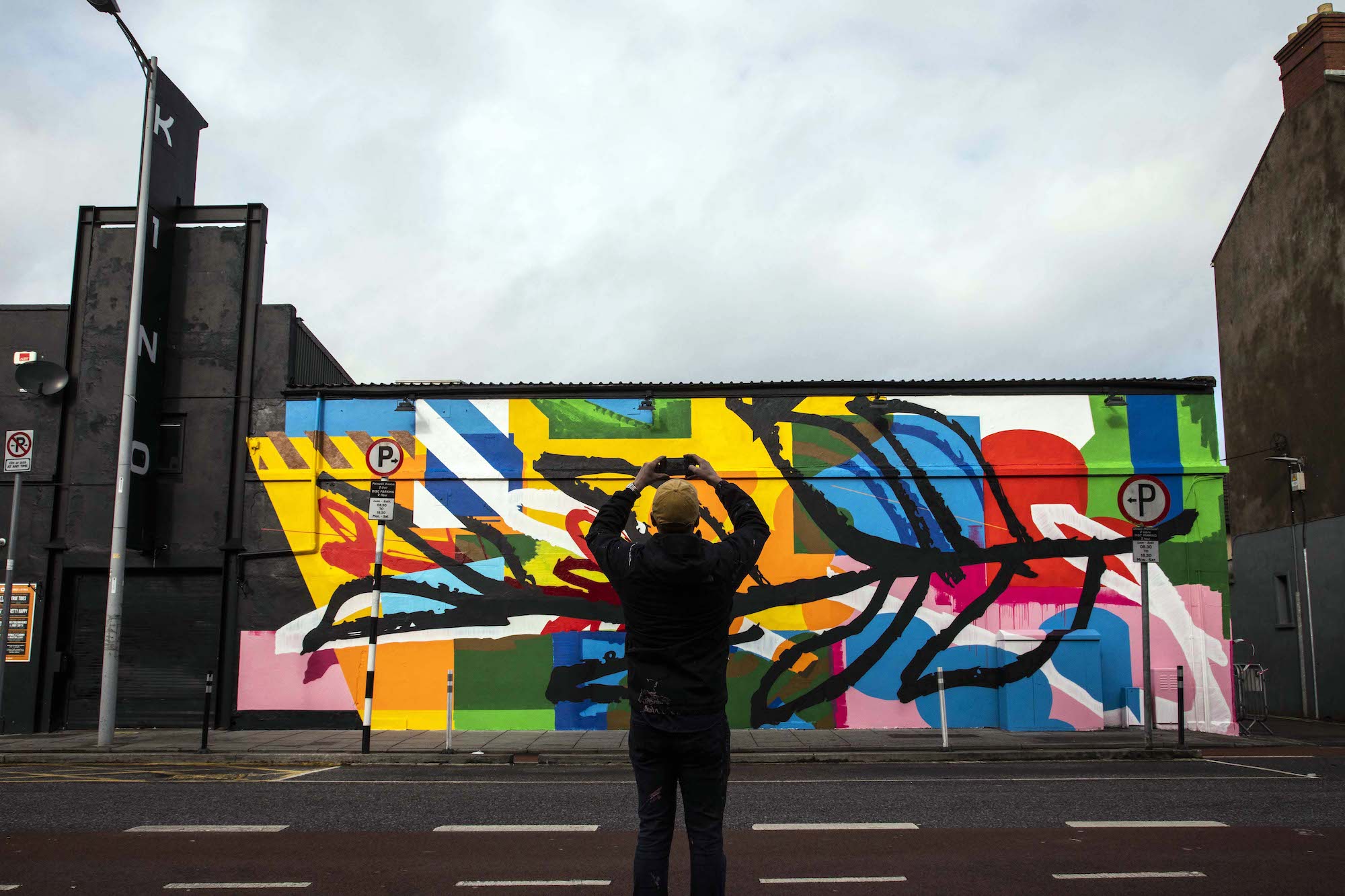In this vivid image, a man dressed entirely in black stands on the side of a wide, at least three-lane road, holding a camera high above his head with both hands. He is photographing a shorter building adorned with a striking, multicolored mural positioned between two taller, plain buildings. The mural, which spans almost the entire length of the building, features an abstract background filled with a vibrant palette of red, blue, green, yellow, pink, white, and black. Dominating the artwork is a black outline of a stem with leaves, resembling a branch, stretching across the mural from left to right. The taller building on the right is brown, while the one on the left, also a multi-story structure, has a large, black poster with white letters spelling out "Kino." The juxtaposition of the richly colored mural against the plain surrounding buildings, along with the man’s posture and attire, creates a striking visual narrative.